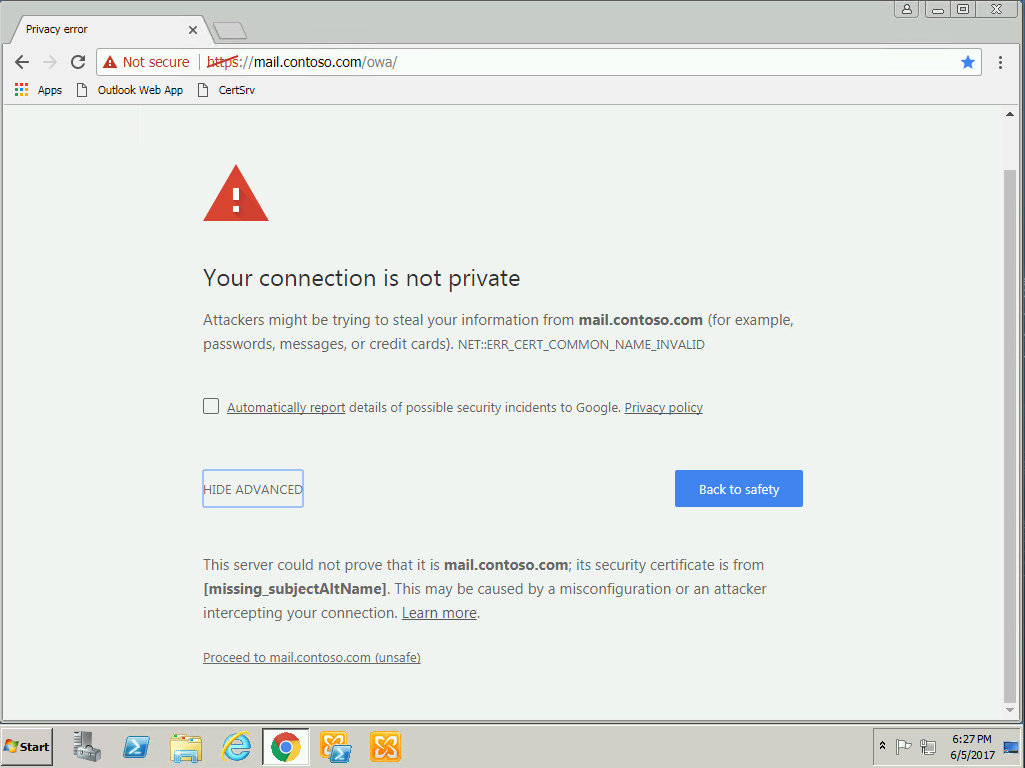**Caption:**

The screen displays a privacy error message on a website, warning the user that their connection is not private. The background is primarily gray, and the address bar prominently shows "Not secure" in red with a red triangle icon, while the HTTPS prefix is crossed out, indicating an issue with the website's security certificate. The website URL is specified as mail.contoso.com.

The main section of the screen features a large red triangle with a white exclamation mark, alongside the message: "Your connection is not private. Attackers might be trying to steal your information from mail.contoso.com (like your passwords, messages, or credit cards)." The URL mail.contoso.com is highlighted in black, emphasizing the potential risk.

Users are given the option to report security incidents to Google via a blank checkbox. Additionally, a "Hide details" link is highlighted with a blue border. A prominent blue button labeled "Back to safety" encourages users to navigate away from the page.

Further details reveal that the server for mail.contoso.com could not verify its identity; the security certificate is missing the subject alternative name. This error might be due to misconfiguration or a potential intercepting threat. A "Learn more" link is underlined, offering additional information. There's also an option to proceed to mail.contoso.com, notably marked as unsafe.

At the bottom of the screen, the taskbar displays various icons, including the Start menu and the File Explorer. The time is displayed as 6:27 PM, and the date is June 5, 2017, in the bottom right corner.